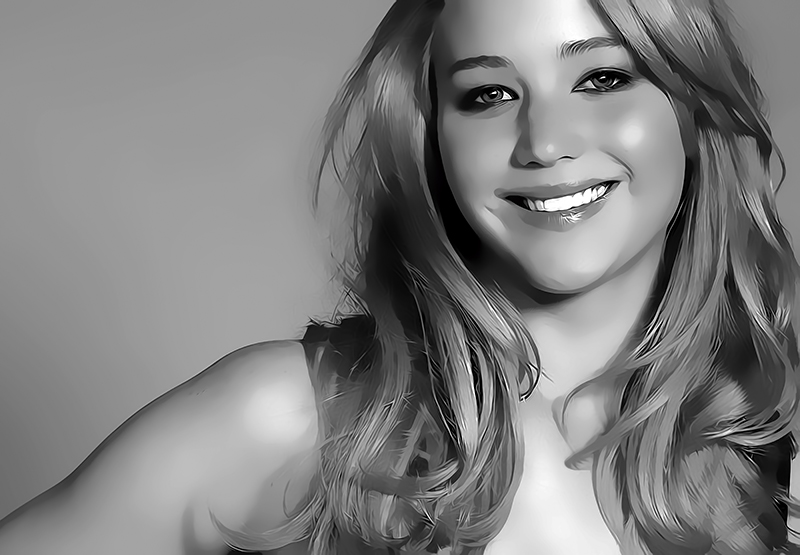This black and white digital painting features a young white woman with wavy, shoulder-length blonde hair cascading over her chest, giving the impression she might be topless although she may be wearing a sleeveless dress. She is set against a plain gray background, smiling directly at the camera with light eyes and white teeth. Her position is centered in the image, which looks digitally produced and lacks any text. The minimalistic composition and grayscale palette emphasize the woman's serene expression and artistic detail.